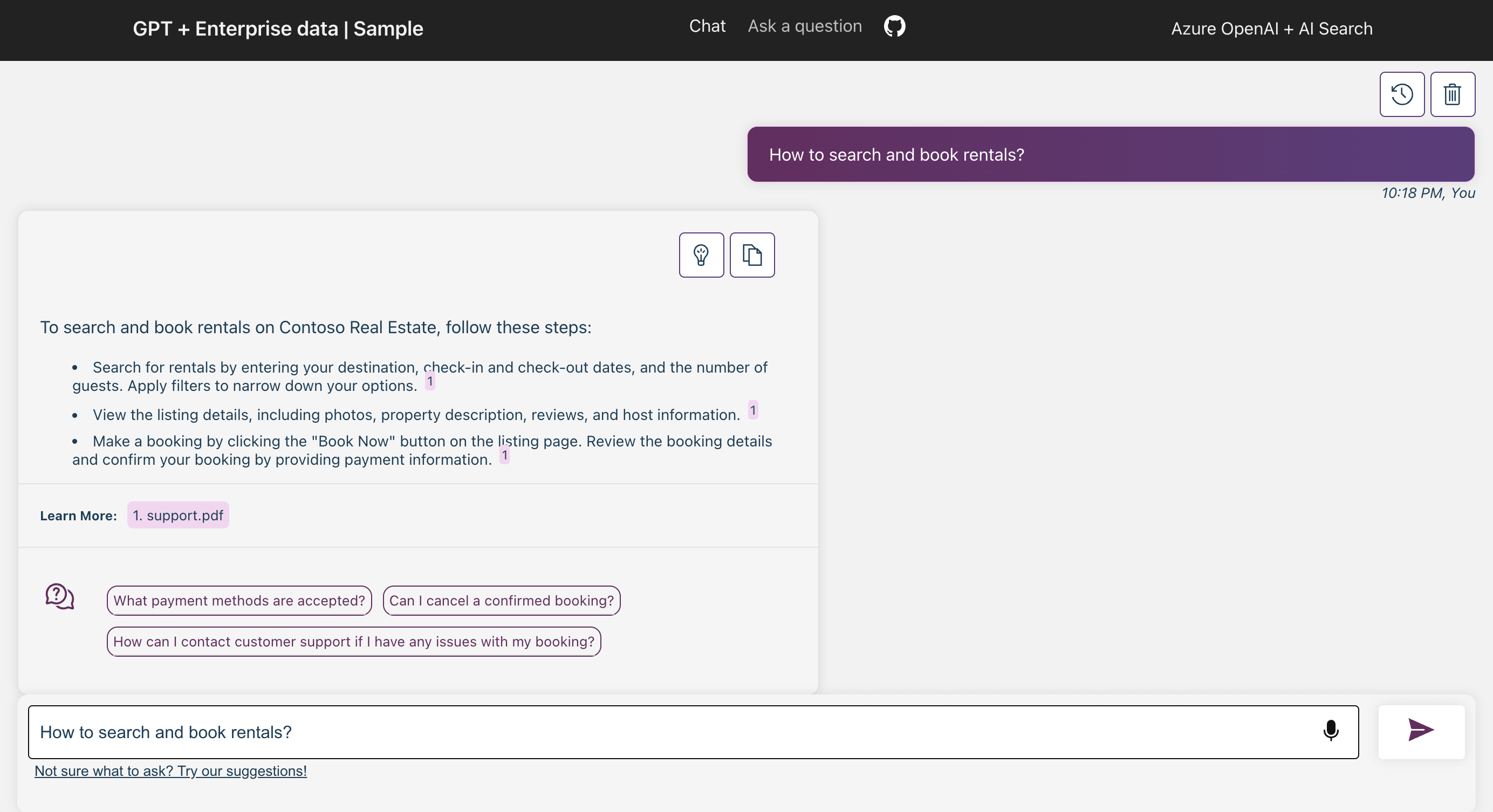This screenshot captures a detailed view of a website designed to assist users in searching and booking rentals. At the very top, there's a black bar displaying "GPT Plus Enterprise Data / Sample." To the right of this text, there are options labeled "Chat" and "Ask a Question," accompanied by what appears to be an icon that resembles either a strand of hair or a GIF of headphones. Further along this bar, you see the labels "Azure OpenAI" and "AI Search."

Immediately below the black bar, there is a bar featuring a clock icon and a trash can icon. Underneath this, a prominent purple bar is titled "How to Search and Book Rentals." Below this bar is a content section containing a small rectangular area on the left side, which includes an icon featuring a light bulb and a piece of paper. This section outlines steps for searching and booking rentals on real estate, formatted with a sequence of steps.

Further down the page, there's a "Learn More" link highlighted pink, which directs users to a PDF file for additional information. Positioned beneath the "Learn More" link are three distinct pink tabs that users can click on to access further details.

Finally, at the bottom of the screen, a bar indicates "How to Search Book Rentals," accompanied by a small purple arrow on the right. This arrow is likely intended for users to click after entering their search query.